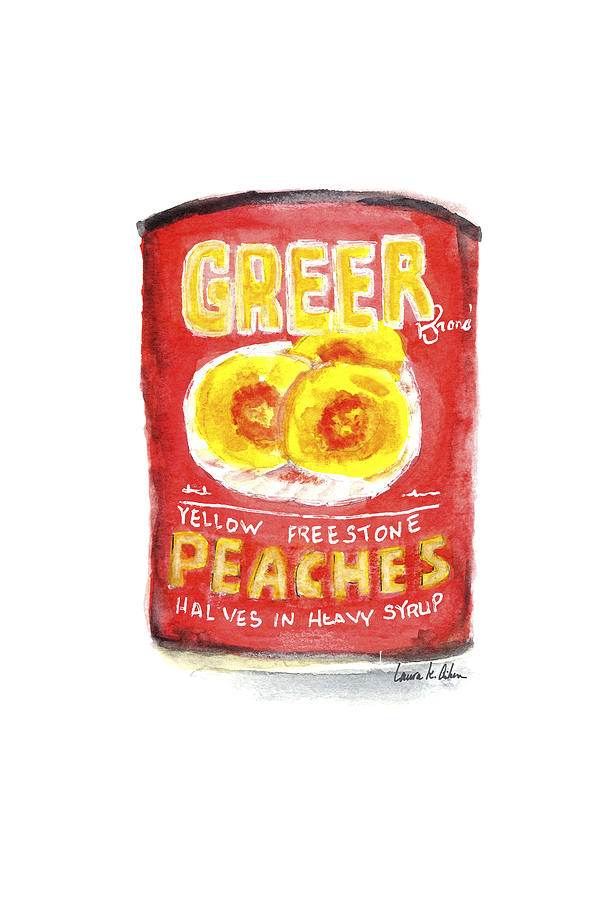This image is an abstract painting representing a red can of peaches. The can prominently features bold yellow lettering that spells "Greer" at the top, with additional text below that reads "yellow freestone peaches, halves in heavy syrup," outlined in white. The design includes three peach halves displayed on a white saucer, emphasizing the peaches' yellowish hue against the red background. The can also showcases the distinctive ridges at the top and bottom, reminiscent of the old steel tin cans. Notably, the artwork is signed by the artist, identified as Laura K. Aiken, near the bottom. Despite its abstract style, the painting clearly communicates the subject and branding details.